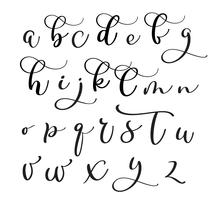The image is an illustration of the alphabet written in a fancy cursive style, consisting entirely of lowercase black letters on a white background. The alphabet is arranged in four rows: the first row displays 'a, b, c, d, e, f, g'; the second row shows 'h, i, j, k, l, m, n'; the third row contains 'o, p, q, r, s, t, u'; and the last row lists 'v, w, x, y, z'. The letters are characterized by their curvy and loopy designs, with some variation in size— most notably the smallest being the 'o' and the largest being the 'y'.